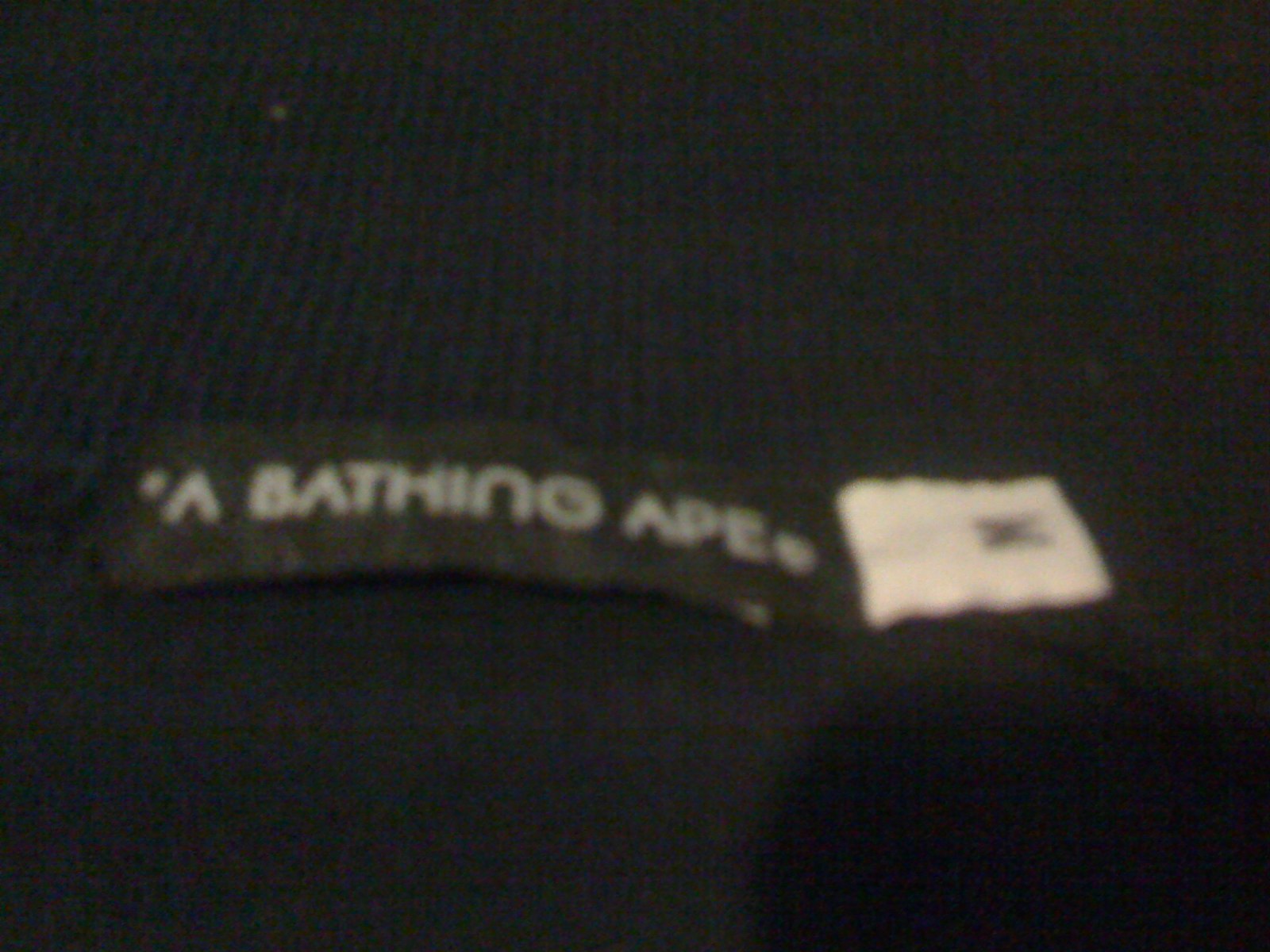This photograph, although extremely blurry and poorly lit, captures a fabric label sewn into a piece of black knit or ribbed clothing. The label itself is also made of fabric and is predominantly black with a smaller white section. On the black portion of the label, the text reads "A BATHING APE," while the white section displays the letter "M," indicating the garment is a size medium. Despite the image's poor quality and lack of clarity, these details are discernible.